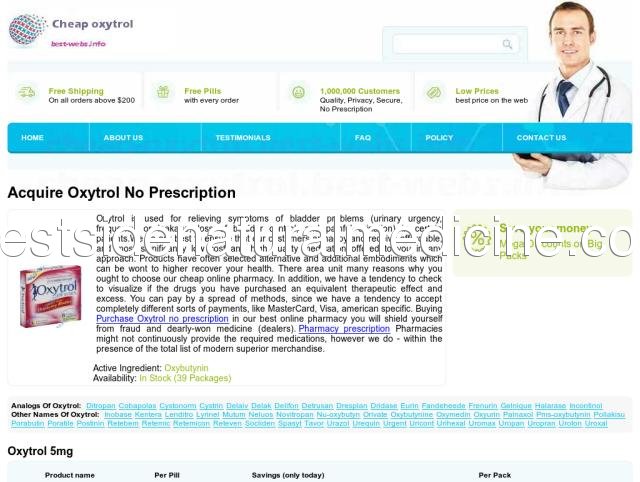The image is a slightly pixelated landscape screenshot, likely captured from a website viewed on a laptop or desktop computer. The website appears to belong to a company named Cheap Oxytrol, which seems to specialize in affordable prescription drugs. The top right corner features a photograph of a young white male doctor, likely in his late 20s or early 30s. He is smiling, wearing a classic white lab coat with a stethoscope draped around his neck, adding a touch of authenticity, though the website's overall design is rudimentary and somewhat unprofessional.

The interface includes several navigational tabs: Home, About Us, Testimonials, FAQ, Policy, and Contact Us. Prominently displayed are several advertisements designed to entice potential customers, including highlights such as "Free Shipping on all orders above $200," "Free pills with every order," boasts of "1 million customers," and claims of "Quality, Privacy, Secure, No Prescription" services. Additionally, the site emphasizes "Low Prices" and "Best Prices on the Web."

The most prominently featured product on the page is Oxytrol, specifically advertised as "acquire Oxytrol, no prescription." Just below this announcement, users have the option to select a 5-milligram dosage. The overall impression is of a basic, slightly outdated e-commerce site catering to those seeking prescription drugs at low prices.